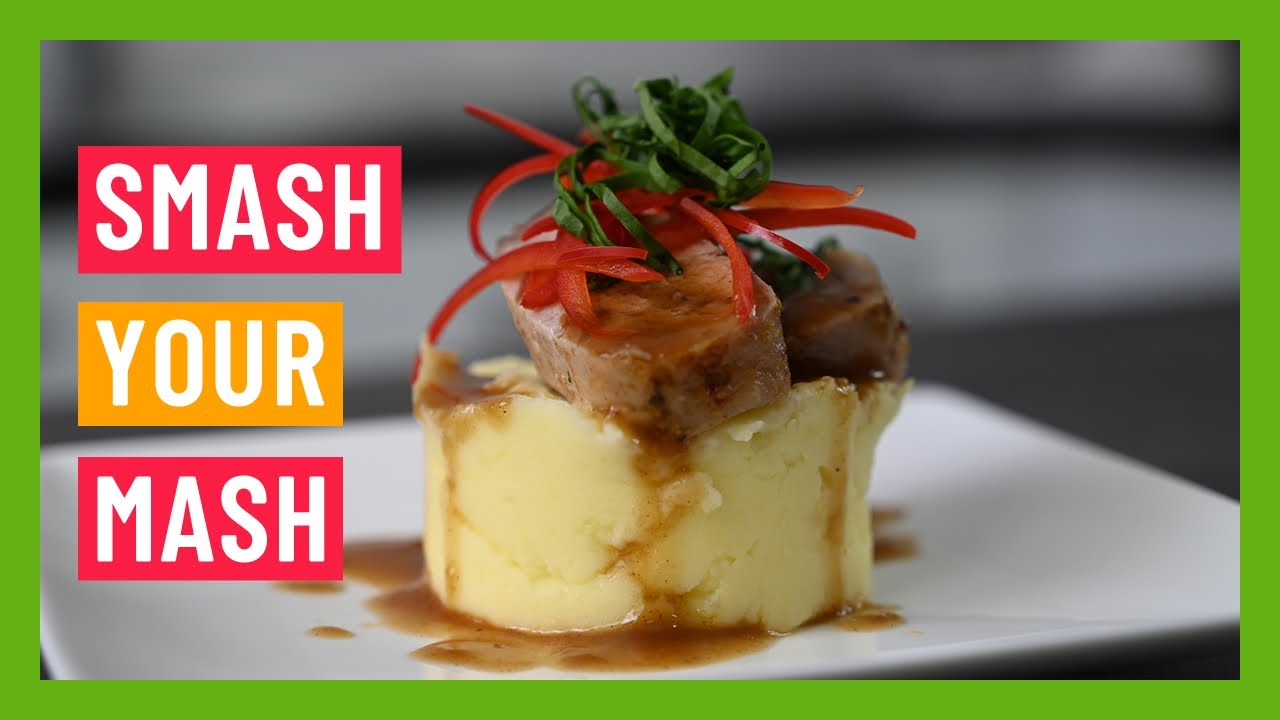This rectangular advertisement features a centrally placed photograph of a culinary dish surrounded by a lime green border. At the left side of the image, bold text reads "Smash Your Mash," with "Smash" and "Mash" inside red rectangles and "Your" within a yellow rectangle. The white square plate in the middle of the photograph showcases a neatly shaped mound of mashed potatoes, topped with two pieces of meat, pickled vegetables, and garnish. A rich brown gravy drizzles over the meat, enhancing the dish's visual appeal. The background of the photograph remains blurry, drawing focus to the intricate and avant-garde presentation of the dish, which suggests it is more of an upscale offering rather than a casual meal.